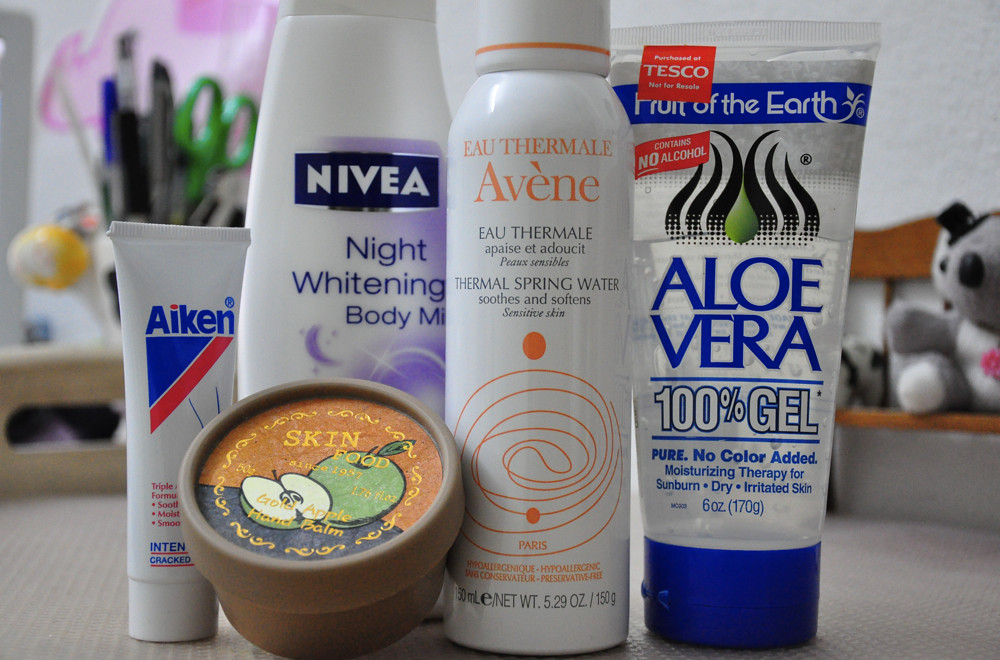This photograph features an assortment of five different skin lotion bottles arranged in a seemingly random manner. The compositions and orientations vary, creating a visually interesting tableau. Let's break down the details:

1. On the far right, there's an aloe vera lotion housed in a transparent container. The bottle has a blue banner near the top and a blue cap at the bottom, although it is positioned upright with the cap resting on the surface.

2. Next, there is a white can labeled "I Have an Egg," distinguished by its white cap at the bottom and a splash of orange on the front. The cap rests flat due to the can’s upright stance.

3. In the center, you find a smaller bottle of Nivea Night Whitening Body Moisturizer. This is a white bottle, with the brand name "Nivea" in navy blue font. It is notably smaller compared to the other bottles and stands with the cap facing downward.

4. Adjacent to the Nivea bottle is another white container with blue accents. It similarly stands with its cap at the bottom, though specifics about its label are less clear.

5. Finally, in front of the Nivea bottle is a small, brown container branded as “Skin.” This bottle, which looks like it is cut in the shape of a fruit, displays an image of a bisected green apple or pear on the front.

In the background of the image, a variety of stationary items are visible. To the right, some pens, markers, and a pair of green scissors can be seen. This contributes to the casual, everyday setting in which this photograph was taken.